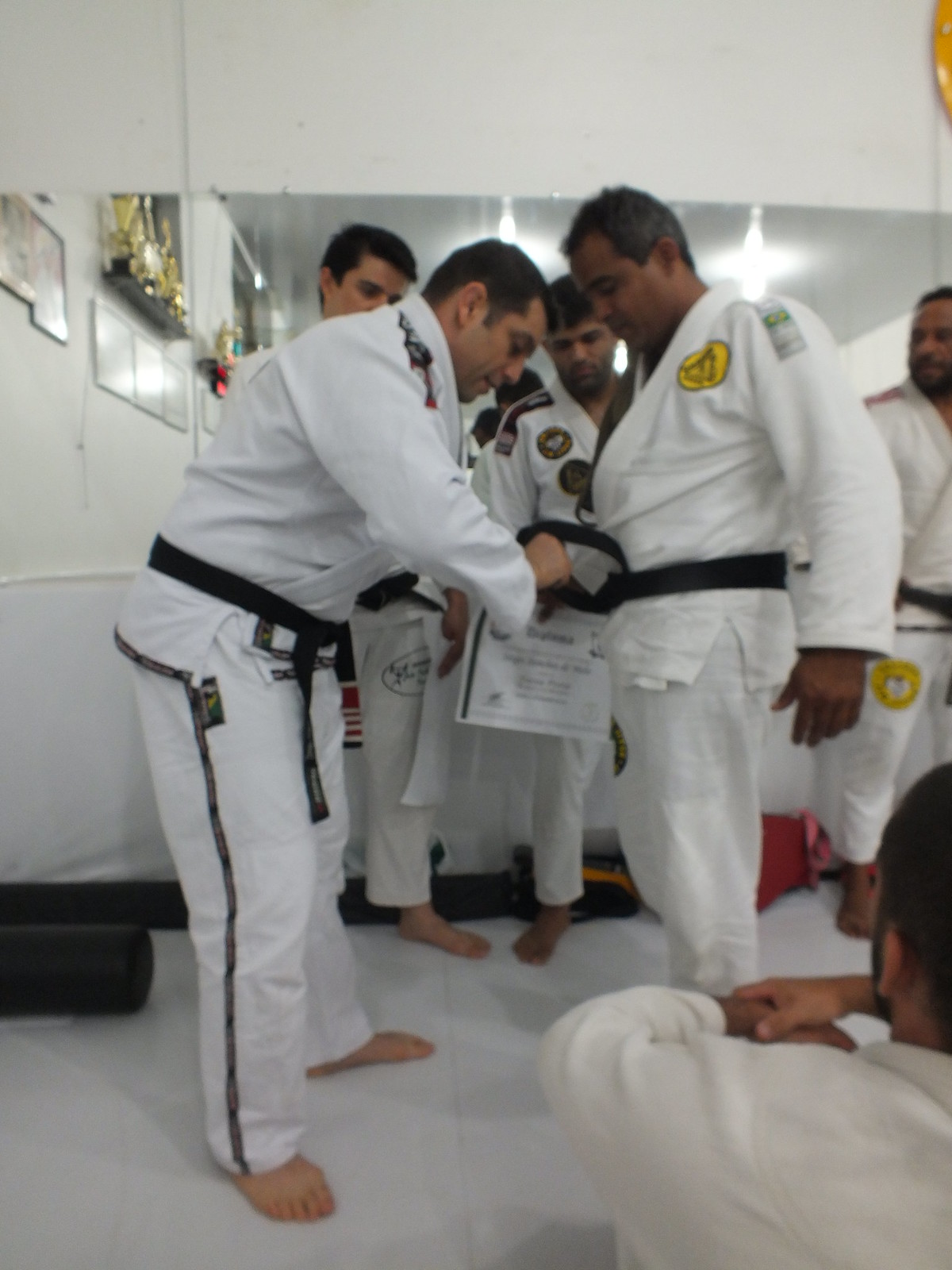The rectangular photograph, seemingly taken inside a dojo, showcases a serene, gym-like space with a white, smooth tiled floor. A large mirror spans the back wall, reminiscent of a dance studio, and the dimly lit room has white walls. The image captures a significant moment involving several men dressed in traditional white martial arts gis, all barefoot. The central focus is on two men: one on the left, bent over, tying a black belt around the waist of the man on the right, who is likely being awarded his black belt. This scene appears to be a formal black belt ceremony, with the man on the left also holding a certificate, presumably to honor the achievement. The remaining men stand by the mirrored wall, observing this pivotal moment, embodying respect and camaraderie while witnessing the special event.